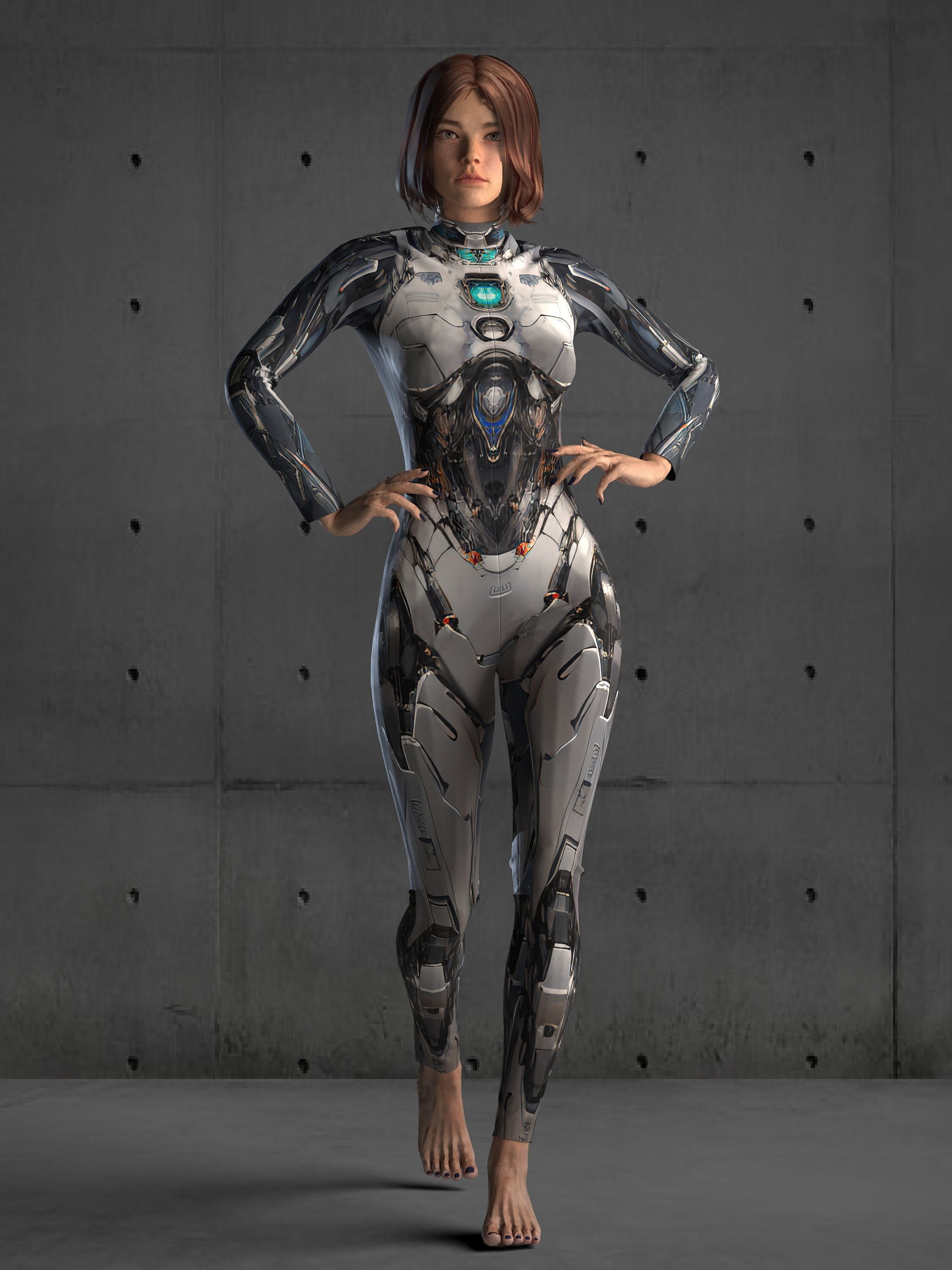The image depicts a highly detailed illustration of a young, feminine robot woman, aged around 20 to 25, with a curvaceous form. She is wearing an intricate, multi-sectioned exoskeleton suit composed of various metals, characterized by its shades of gray and dark gray. Embedded in the exoskeleton, several lights shine through—the most prominent being a green light emanating from her chest and a bluish light atop the suit. The robot woman has short, brunette hair and exhibits a fair, caucasian skin tone. She stands barefoot with her right foot slightly raised off the ground, hands on her hips, and a neutral expression on her face. The background is an industrial gray room featuring a symmetrical pattern of tiny, bolt-like dots on the walls and matching gray flooring, enhancing the futuristic and mechanical ambiance of the scene.